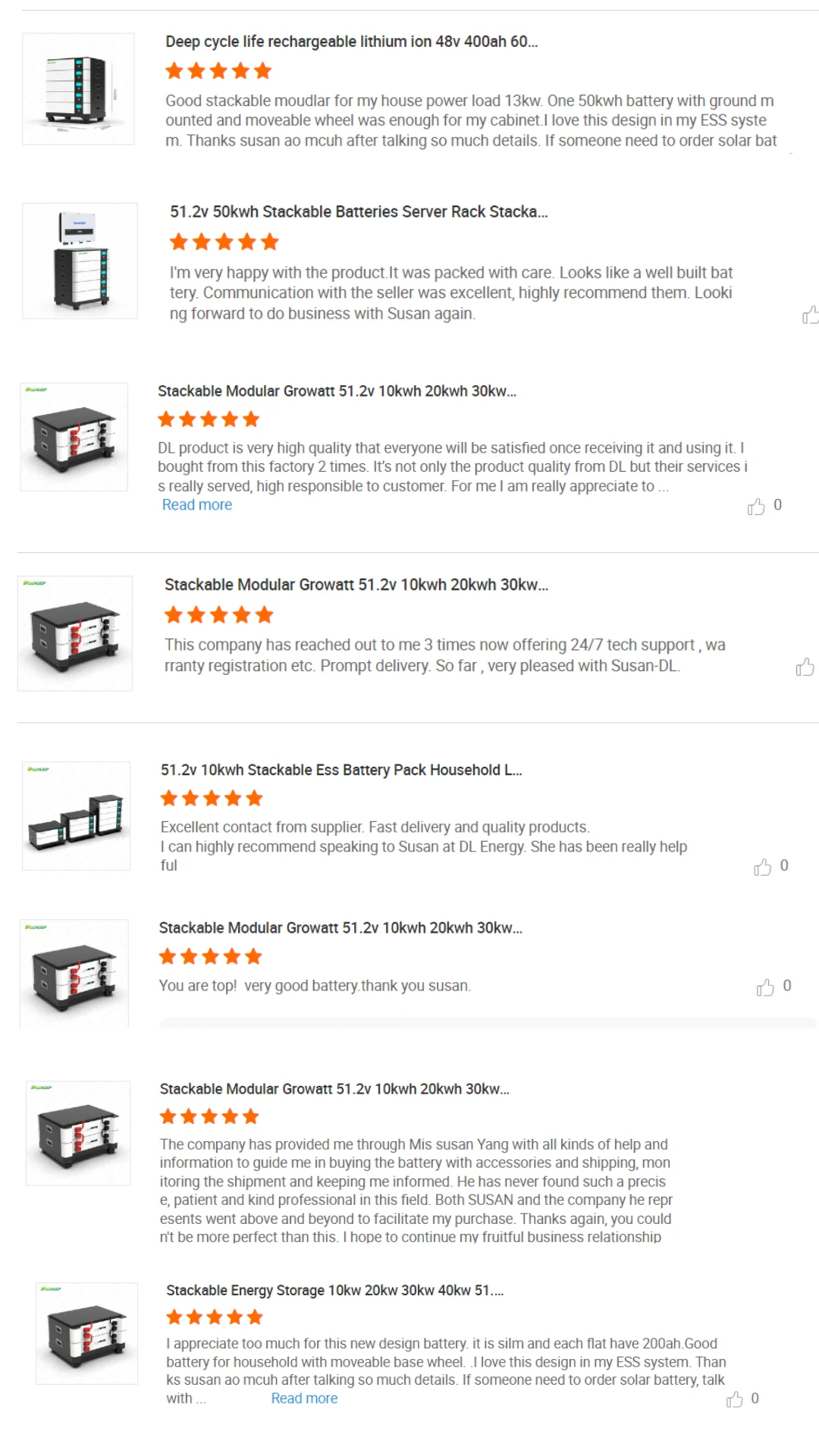The image depicts a lineup of various high-performance battery rack servers, meticulously organized to highlight their features and specifications. At the top of the image, a highly-rated, five-star, deep cycle life rechargeable lithium-ion battery is prominently displayed. This model operates at 48 volts and is designed for stackable configurations. 

Below this, a versatile and portable battery rack system is showcased. It boasts a 51.2-volt capacity and an impressive 50-kilowatt-hour energy storage capability, emphasizing its stackability and efficiency in power management.

The subsequent row features a low-profile, stackable, modular battery system branded as Growatt. Another identical Growatt unit is positioned adjacent to it, underscoring the modular and scalable nature of these batteries.

Further down, three battery packs are presented side by side, varying in size from small to medium to large. Each of these units is classified as a 51.2-volt stackable ESS (Energy Storage System) battery pack designed for household use, offering flexible energy solutions depending on the user’s needs.

The bottom section of the image showcases several more Growatt battery systems, consistently maintaining the same stackable and modular design. Like their counterparts above, these units have also received five-star ratings, indicating their reliability and high customer satisfaction on the platform where they are listed.

Overall, the image serves as a comprehensive display of cutting-edge, stackable battery systems, ranging in size and application, all praised for their performance and dependability.